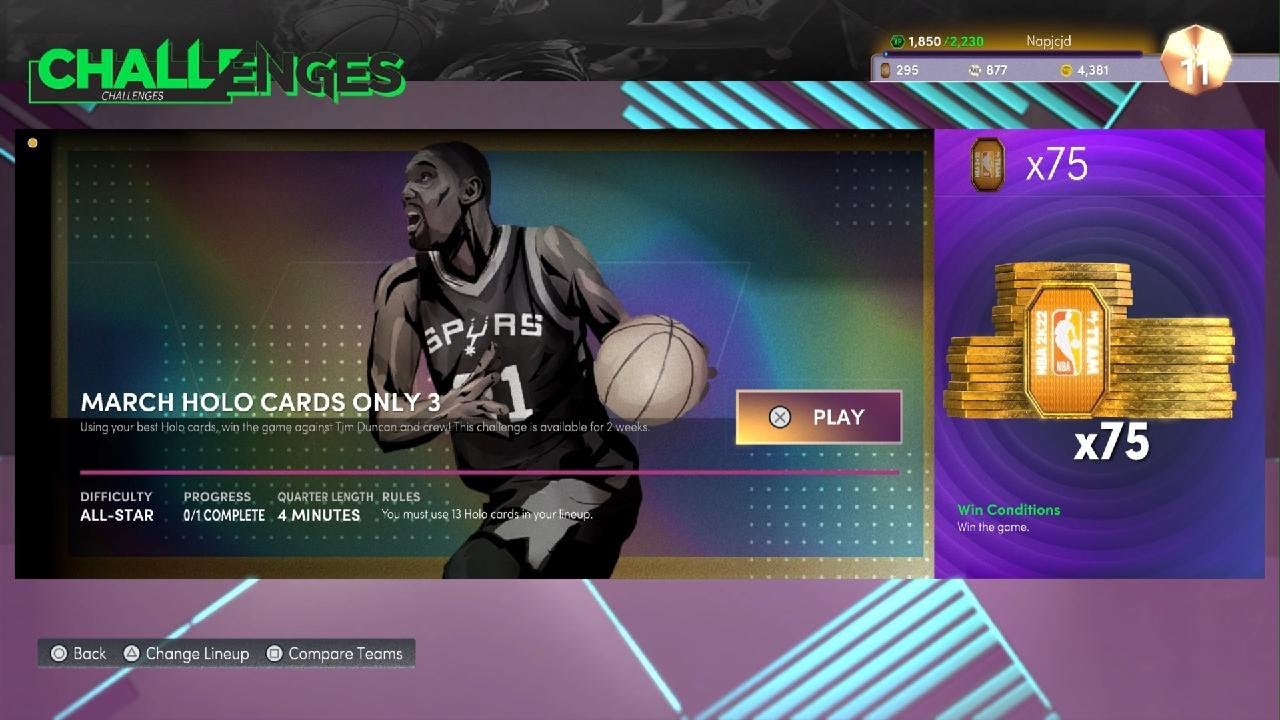**Detailed Caption:**

This image, categorized under Websites, showcases a dynamic and vibrant interface. A marble-like bar stretches across the top in a sophisticated black-and-white design. Prominently displayed in bold green and black letters is the word "Challenges." Centered at the top of the bar is a time range, "1500-2230." The frame of the interface is highlighted with a purple border, accentuated by intermittent teal lines.

At the top center, there is a notable gold coin icon embossed with the number "11". In the background, an intense basketball player is depicted mid-action, carrying a ball in his left hand while his gaze is directed upwards. Above this image, the text reads "March Holo cards only 3," followed by "Difficulty All Star" and "Progress 01 Complete". Further details mention the "Quarter length rules: 4 minutes."

Below this informative section is a prominently placed "Play" button, while a "Back" button is located further down. Additional options to "Change line up" and "Compare teams" are available.

To the right side of the interface, win conditions are specified with "Times 75," illustrated by an image of a pile of gold ticket-like objects. The entire lower portion features a purple background adorned with sporadic teal lines.

The basketball player’s background adds a dynamic flair with a swirly pattern of multicolored hues, including orange, purple, and blue, enhancing the vibrant and engaging feel of the interface.